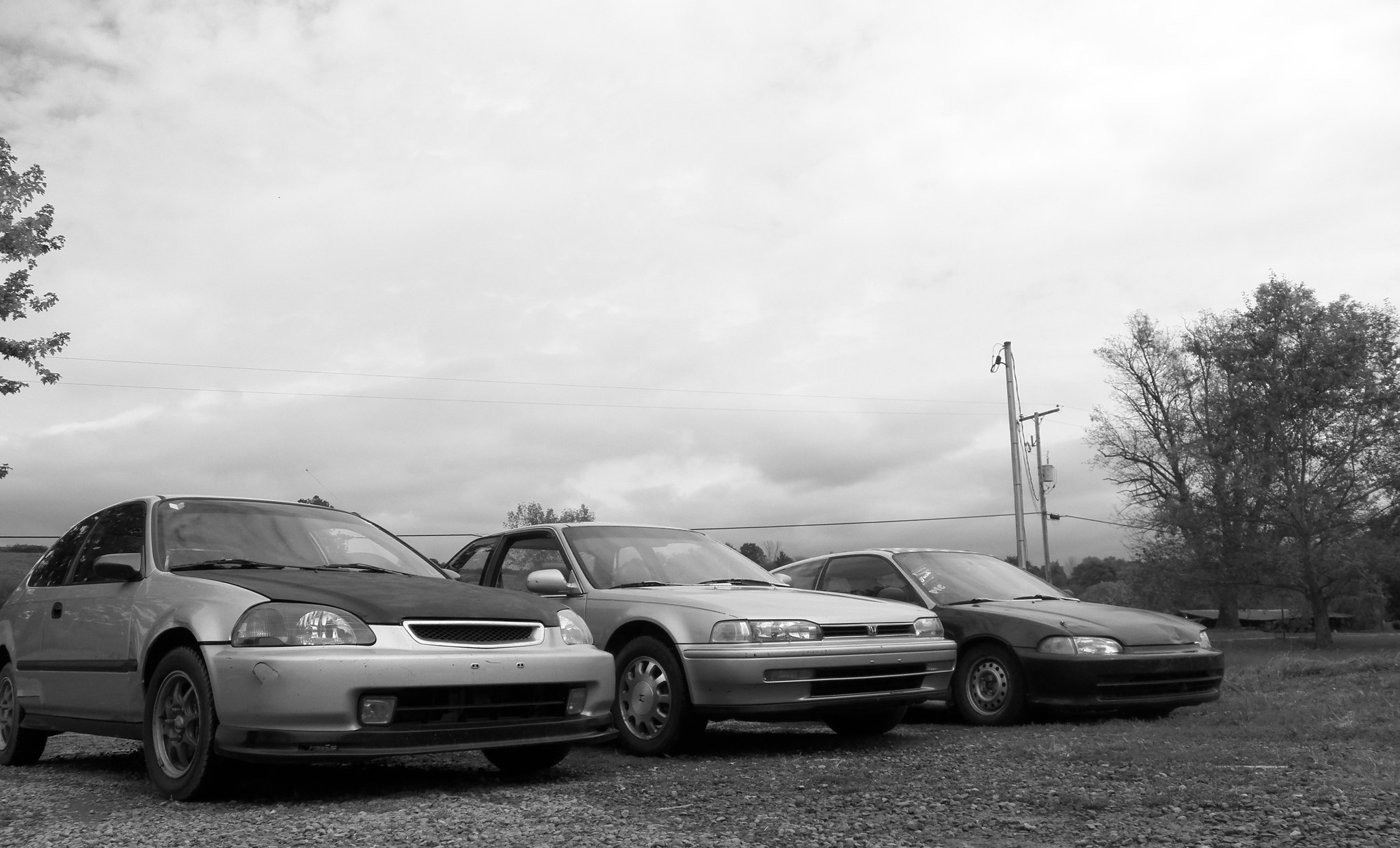This black-and-white photograph captures a trio of small sedan-type vehicles parked in a line on a dirt surface with patches of grass visible on the right edge. The cars are viewed from a low-angle, front perspective, closely aligned from the bottom left corner towards the middle right. The car on the left is distinctive with a darker hood than the rest of its body, which is a lighter, uniform color. The middle car appears to be a light, solid color, while the car on the right is uniformly dark. The overcast sky occupies the top part of the image, casting a gloomy light over the scene. In the backdrop, there are several trees—two on the right and one partially visible in the upper left. An electrical pole with a line runs parallel to the cars, adding an element of industrial contrast to the natural and automotive setting.